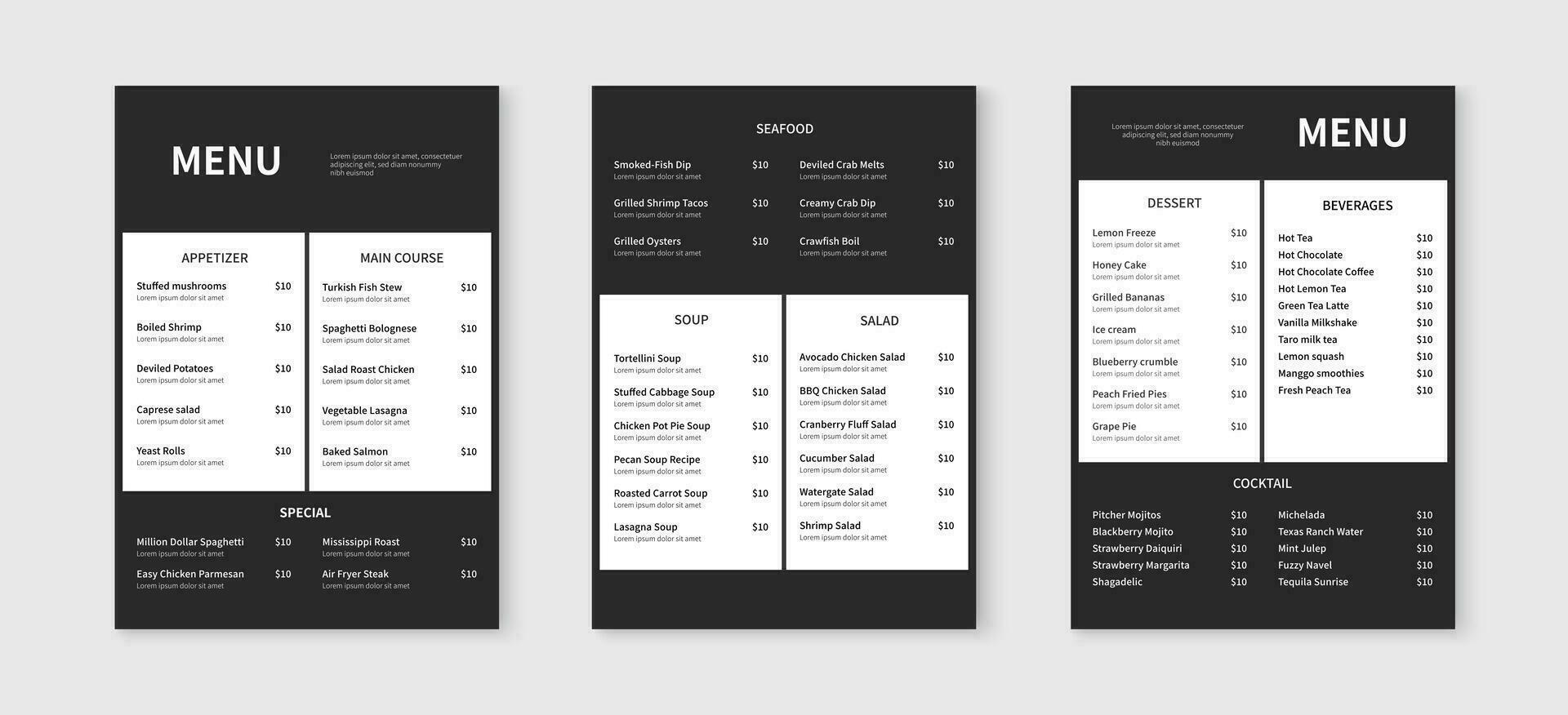The image showcases a detailed restaurant menu, presented in three distinct pages laid horizontally on a gray surface. Each page is designed in black and white, emphasizing a professional aesthetic. The first page, with a black background, features two white boxes labeled “Appetizers” and “Main Course,” followed by a section for “Specials” at the bottom. The second page similarly contrasts with a black top section labeled “Seafood,” followed by white boxes for “Soup” and “Salad.” The third page contains white boxes listing “Desserts” and “Beverages,” with “Cocktails” detailed in a black section at the bottom. Highlighted dishes include stuffed mushrooms, boiled shrimp, deviled potatoes, and million dollar spaghetti. Notably, everything on the menu is priced at $10. The uniform design across the three pages uses white text on black sections for clarity, ensuring the categories and items stand out.